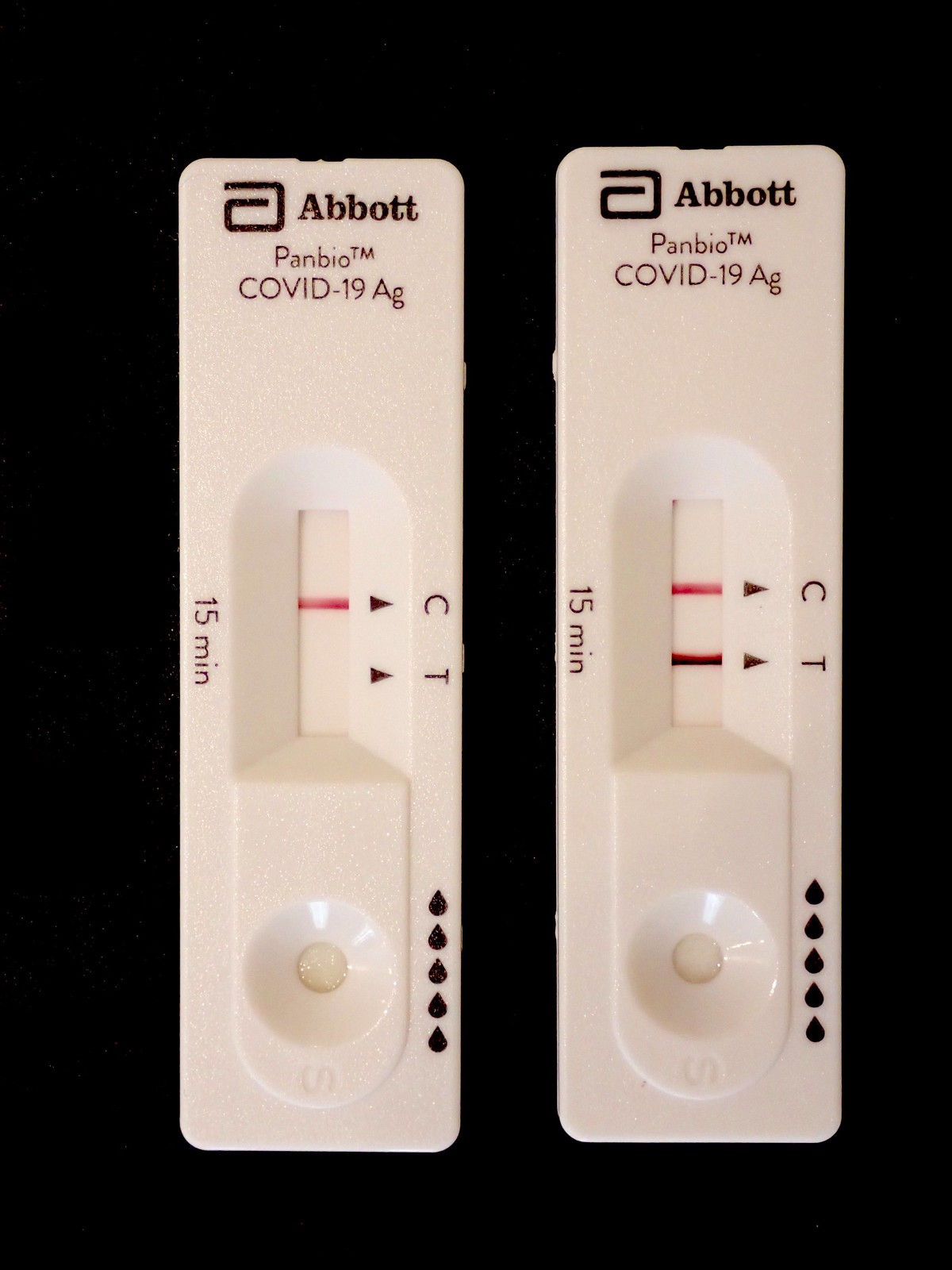The image showcases two COVID-19 test kits positioned side by side against a black backdrop. Each test kit is a long rectangle, oriented vertically. At the top of both kits is the "Abbott" logo, accompanied by a distinctive emblem resembling a backwards capital "G." Below the logo, the kits are labeled "Panbio™ COVID-19 AG."

Each test contains a vertical rectangle window centrally located, featuring a red line approximately 60% from the bottom. Beside each red line is a right-facing arrowhead and the letter "C," both oriented downwards. Below this, the letter "T" appears, accompanied by another arrowhead pointing towards it from the left.

On the far left side of each test, the text "15 min" is written vertically downwards. At the very bottom of each test, there's a small circle encircled by an outward circle, resembling a flat funnel with the center being the lowest point. Adjacent to this feature are five black drops, aligned vertically.

The first test kit displays a single red line beside the "C" in the window, indicating a negative result. The second test kit, however, has two lines: a red line beside the "C" and another red line accompanied by a black overlay beside the "T," indicating a positive result.